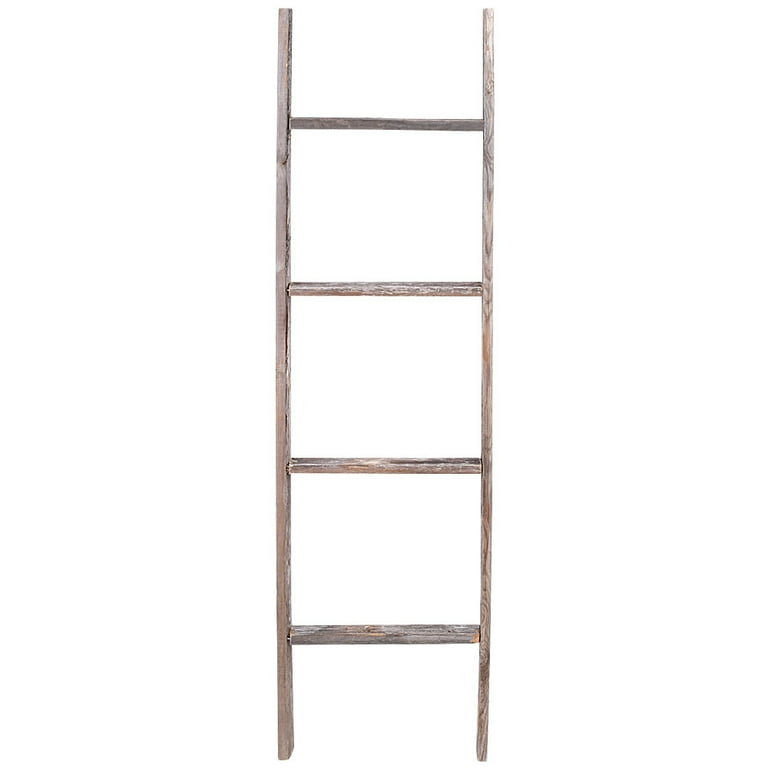This is a color photographic image of a wooden ladder placed against a plain white background. The ladder features four horizontal rungs—one, two, three, four—suggesting its limited height, although its exact size is difficult to determine due to the lack of contextual clues or points of reference in the photograph. It is crafted from pale, weathered wood with varying shades of light brown and gray, indicative of age and frequent use. The vertical poles running up either side of the ladder appear a bit smoothed out, minimizing the risk of splinters. Notably, the topmost part of the left pole is slightly white, and closer inspection reveals subtle cracks in the wood grain, especially on the left-hand side. The photo depicts the ladder as a free-standing object, centrally positioned without any additional elements or text.